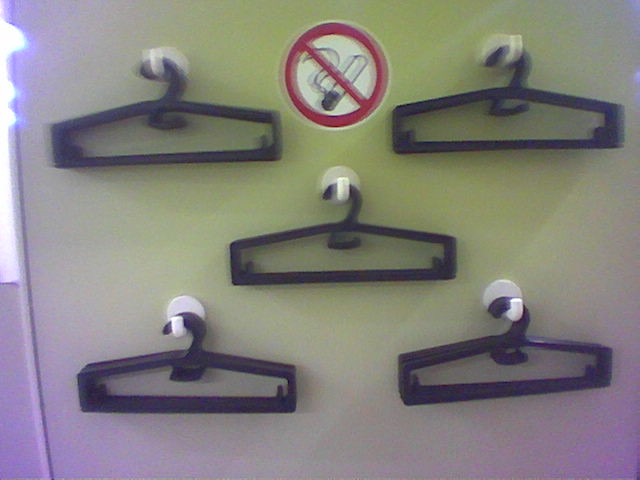This slightly blurry photograph depicts five black plastic clothes hangers suspended from five white command hooks against an off-white wall. The hangers have a distinctive pentagonal shape with straight sides and tiny black upward-pointing hooks. The wall appears off-white but is tinged with a slight green hue at the top and purple along the edges and lower side due to the lighting in the room. A light source is visible at the very top left of the image, casting subtle shadows. Central to the arrangement, towards the upper center, a red "No Smoking" sign is prominently displayed. This sign features a red circle with a diagonal red slash from the upper left to the lower right, crossing over a black and white image of a lit cigarette with a brown end and swirling smoke. The hangers are positioned as follows: one on the upper left, one to the upper right adjacent to the "No Smoking" sign, one directly below the sign in the middle, one on the bottom left, and one on the bottom right.